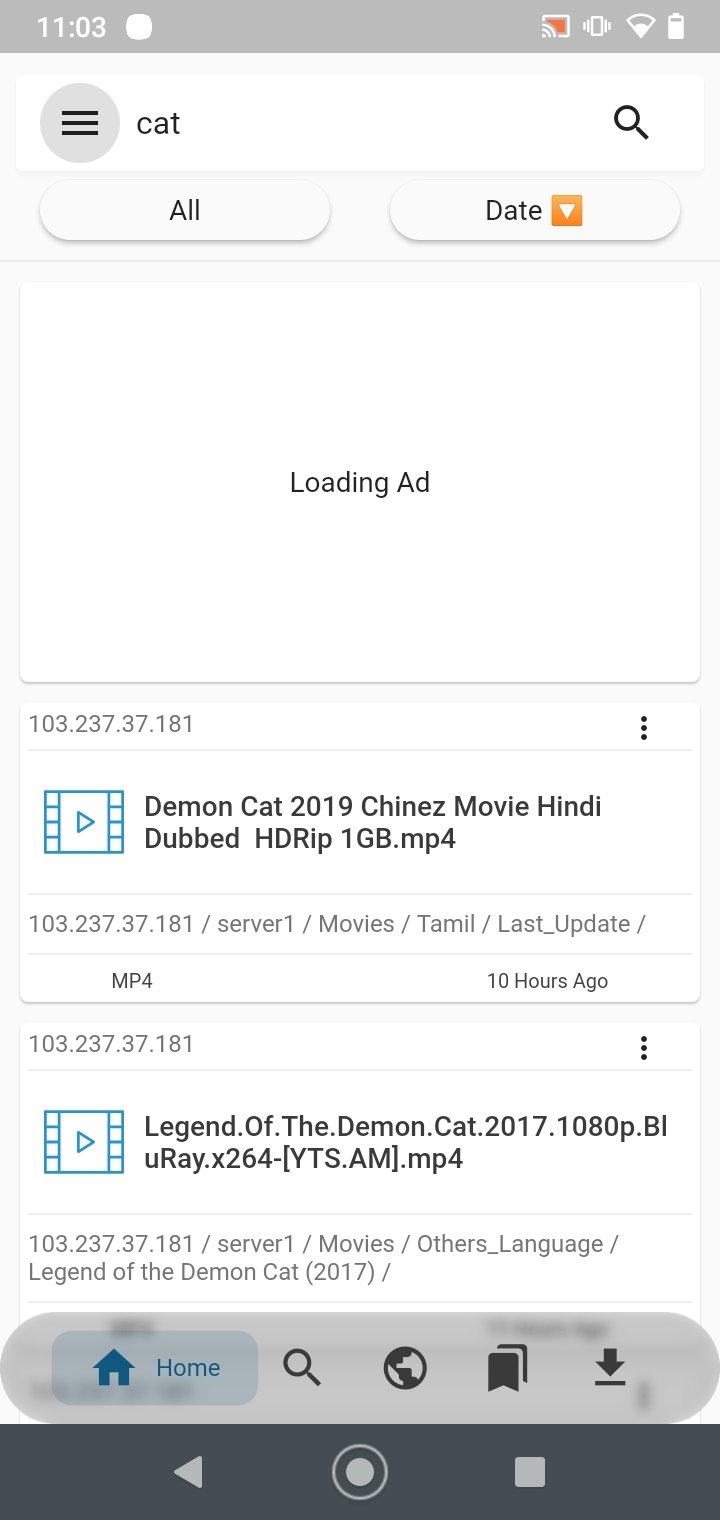**Descriptive Caption:**

A vibrant, color screenshot captured at 11:03 AM showcases a smartphone's interface at 80-90% battery life with a weak connection. The display reveals a search result for "cat" on an unspecified app, with an active ad loading at the top, currently visible only as a blank white area with the text "loading ad." Below the ad section, two search results appear. The first is "Demon Cat 2019," a Chinese movie dubbed in Hindi, with a file size of one gigabyte and listed server information. The second result is "A Legend of the Demon Cat 2017," also accompanied by its server details. The first movie was uploaded 10 hours ago. At the bottom of the screen, the navigation bar includes a back button, a home button, and an option to download the videos.